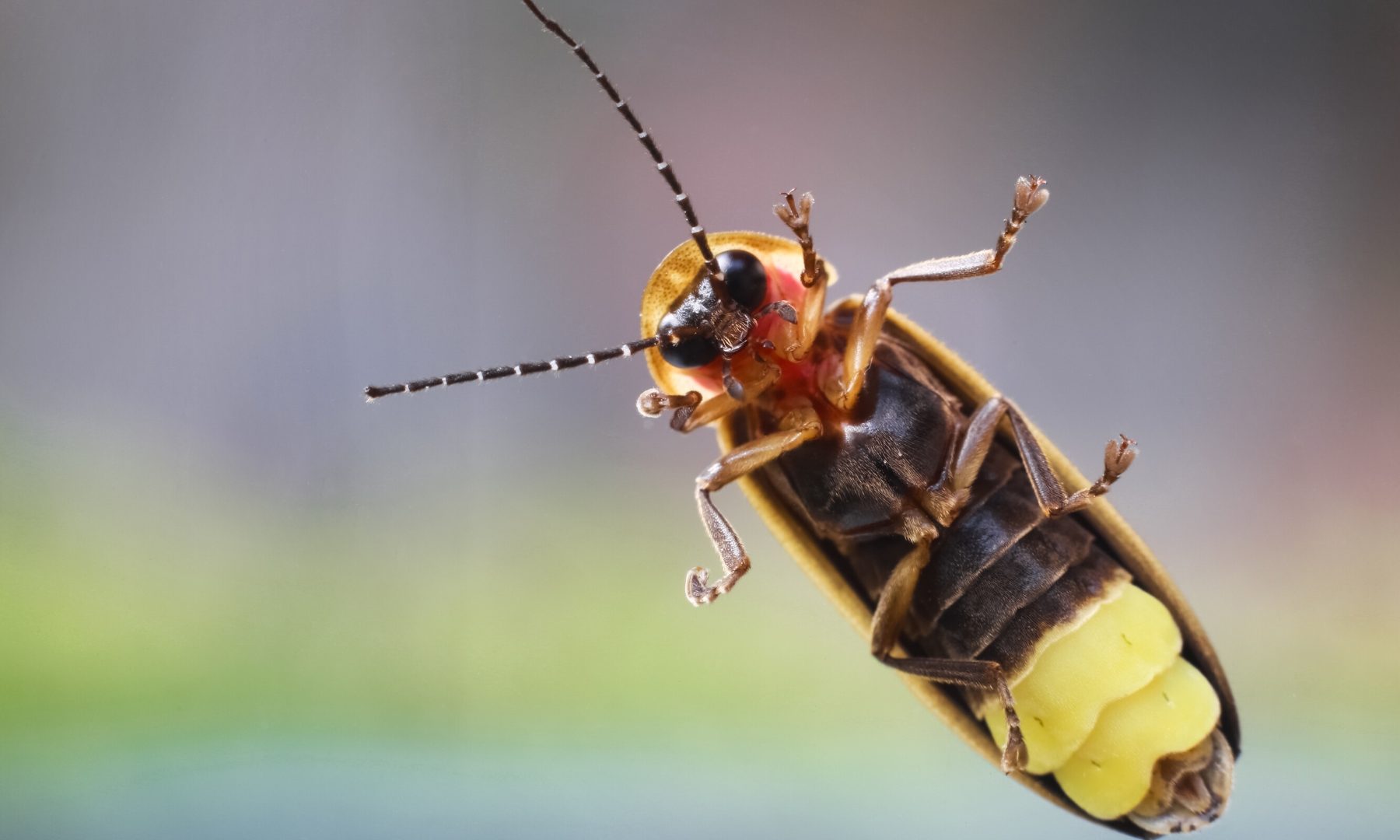This image is an extreme close-up photograph of the underside of a beetle, showcasing intricate details of the insect's anatomy. The beetle's exoskeleton is prominently visible, with a predominantly brown body transitioning to a vibrant yellow near the tail end. The beetle has six legs, with the first pair being notably shorter than the remaining four, which are bent while the front pair extends straight downward. The legs exhibit a silvery brown hue. The beetle's face features large, dark eyes and long, black antennae adorned with distinctive white stripes or bubbles. Additionally, there is a red tint under its chin and around the bottom of its eyes. The insect’s head is sheltered by a section of its outer shell. The background is artistically blurred with a mix of green, light blue, and purple hues, emphasizing the beetle's detailed underbelly.